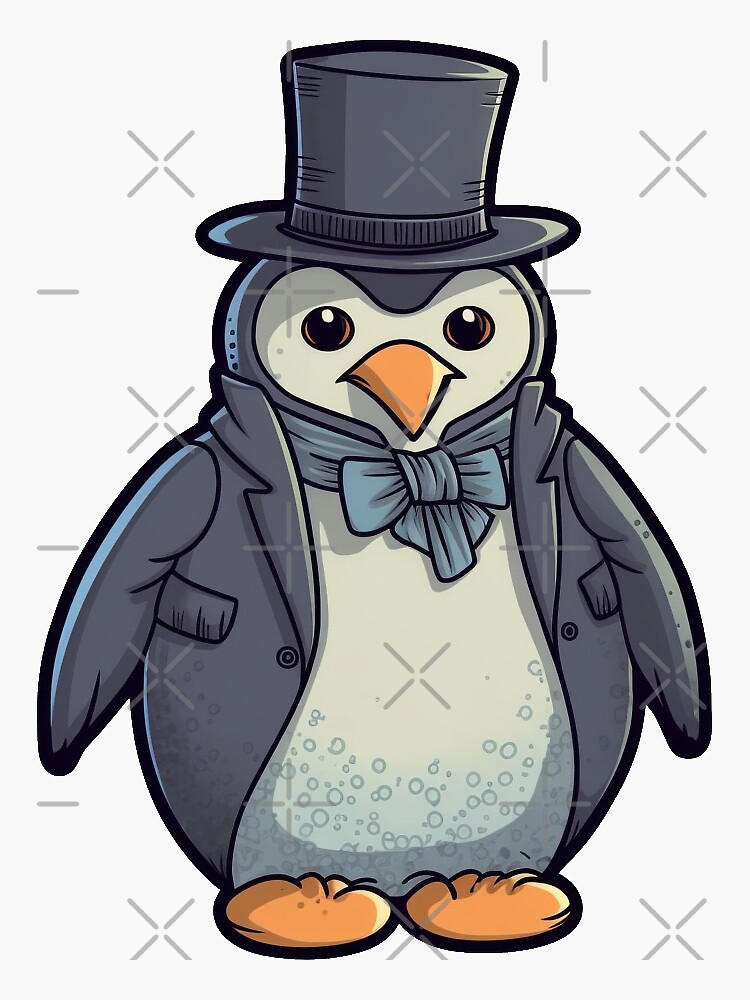The image is a computer-generated, cartoon drawing of a penguin dressed in formal attire. The penguin features a black overcoat, matching the dark gray of its natural coloring, complete with pockets and buttons. It wears an elegant black top hat and a blue neck scarf tied into a bow tie. The penguin has a white face and belly, yellow-orange feet, and a yellow-orange beak. The background is white and includes a subtle light source emitting a blue hue on the penguin's right side (left side of the image). There are distinctive watermarks over the image, composed of X shapes, plus signs, and dashes, typical of stock photos. Additional details include multiple circles along the bottom part of the penguin's coat.